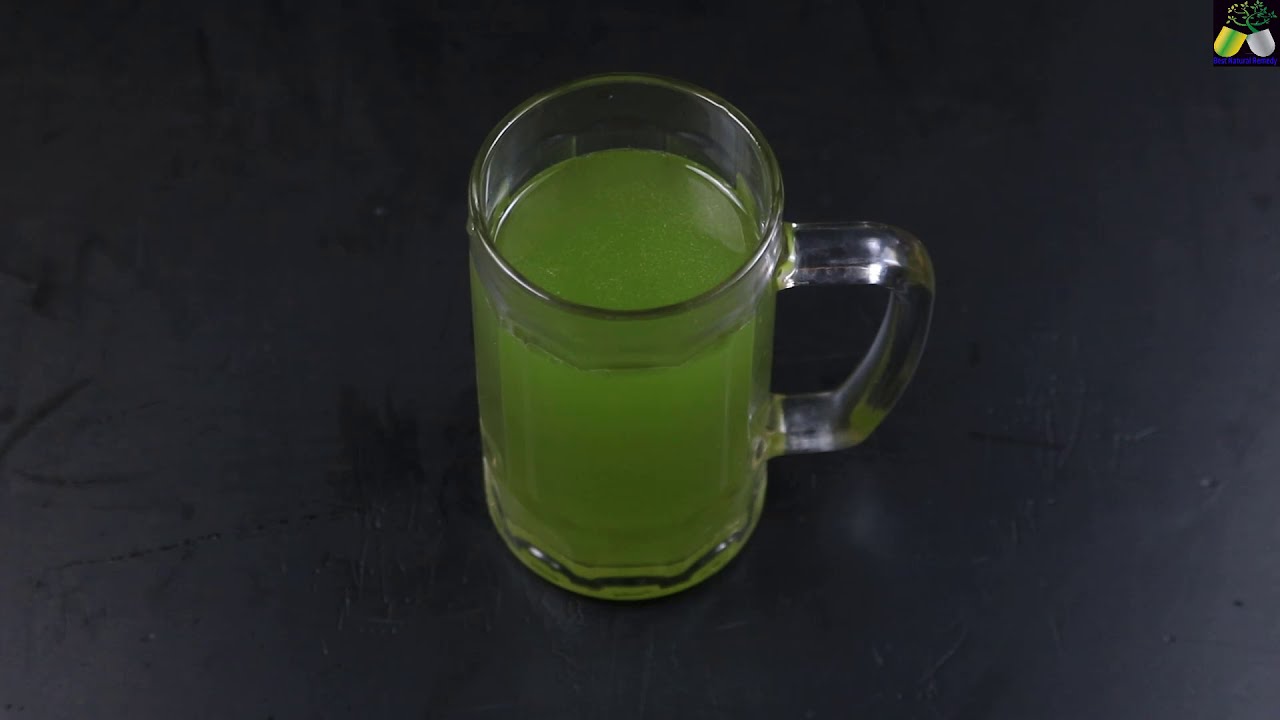An up-close, slightly elevated view of a clear glass mug filled about 7/8 of the way with a bright lime green liquid. The mug, positioned centrally, has a handle projecting to the right. It sits on a black, somewhat dusty table which resembles a lab tabletop. The background is stark and devoid of any other objects or text. In the upper right-hand corner of the image, a small logo is visible. The logo consists of two halves: the left side featuring green and yellow elements and the right side in gray. Above these are squiggly white lines, possibly representing a branding motif. The logo is distinctive yet unclear, resembling broken capsules or possibly vases, with some suggesting it includes a hint of a plant-based design.